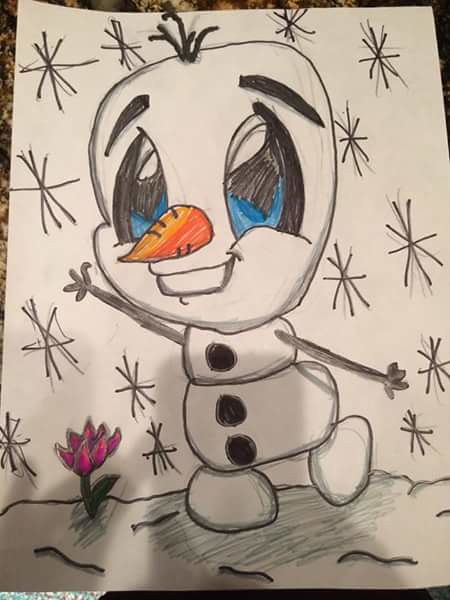In the photograph, a piece of white drawing paper is laid out, showcasing a lively and cheerful hand-drawn snowman. The snowman's body is composed of two snowballs, adorned with three black buttons in the center. Its head features expressive details: blue eyes, thick eyebrows, and a tuft of hair peeking at the top. Adding to its cheerful disposition, the snowman has a wide smile and a distinctive carrot nose. It extends its arms in a wavy gesture, enhancing its jovial demeanor.

On the ground beside the snowman, a vibrant red flower with a winding green vine stands out against the snowy backdrop. Snowflakes gracefully fall from above, contributing to the wintry scene, while a layer of white snow blankets the ground. The entire drawing is set on a table, with the subtle shadow of the photographer faintly visible on the paper, adding a personal touch to the captured moment.